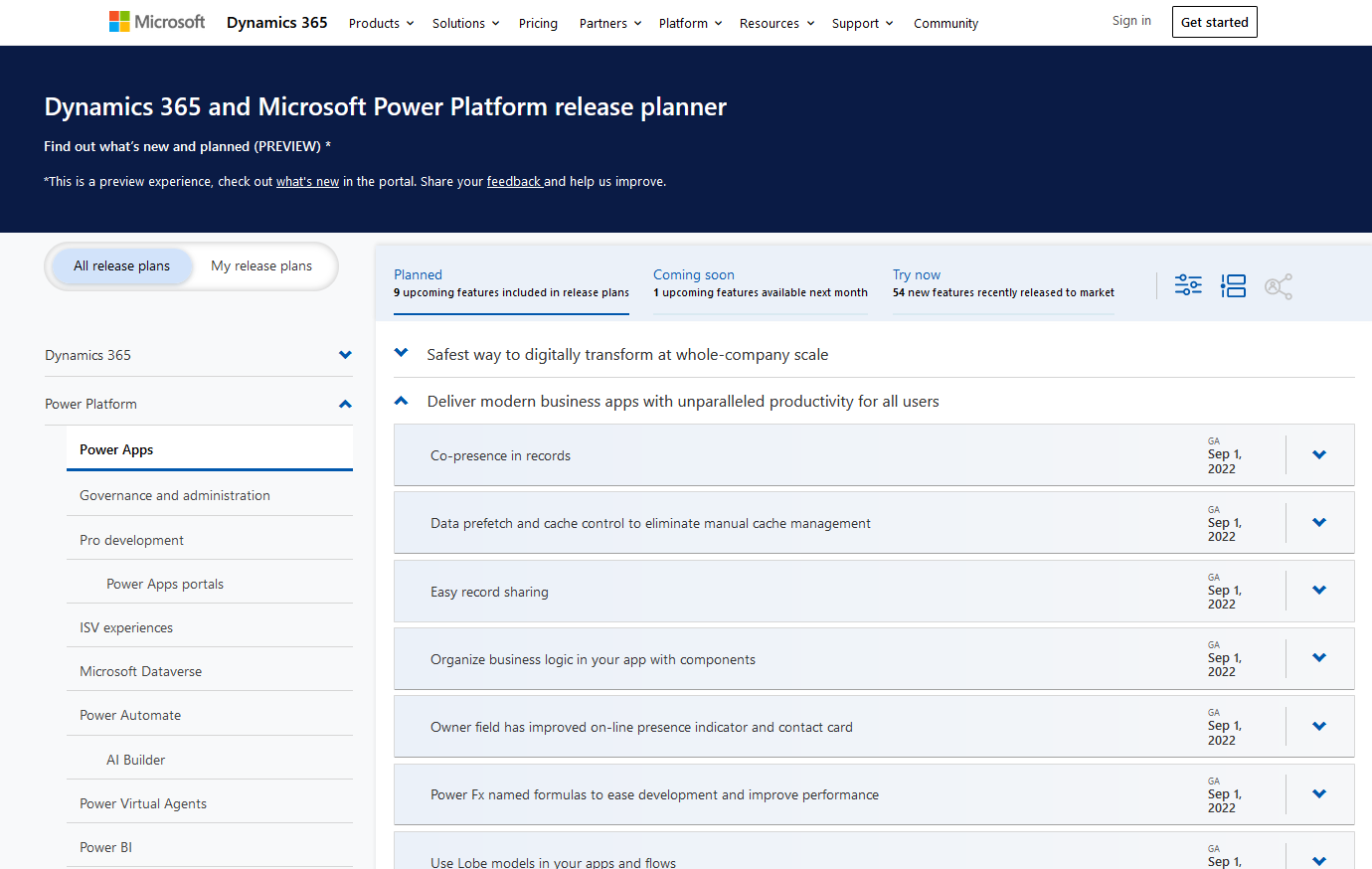The image is a screenshot from the Microsoft Dynamic 365 and Power Platform Release Planner interface. The top navigation bar displays various menu options starting from the left, including products, solutions, pricing, partners, platform, resources, support, and community—each accompanied by a dropdown arrow for further options. On the right side of the navigation bar, there are 'Sign In' and 'Get Started' buttons within a highlighted box.

Beneath the navigation bar, there's a prominent blue strip with white text announcing "Dynamics 365 and Microsoft Power Platform Release Planner" and an invitation to "Find out what's new and planned." The term "preview" appears in parentheses next to this phrase, accompanied by an asterisk, which leads to a note below stating, "This is a preview experience." The strip also contains links to "Check out what's new" and "Share your feedback," both underlined for emphasis.

Below the blue strip, the interface is split into two main sections. On the left, a sidebar provides navigation for "All release plans" and "My release plans." This section includes a dropdown menu for Dynamics 365 and an expanded menu for Power Platform, listing subcategories such as Power Apps, Governance and Administration, Pro Development, Power App Portal, Integrated App Service (IASB) experience, Microsoft Dataverse, Power Automate, AI Builder, Power Virtual Agents, and Power BI. In this list, "Power Apps" is highlighted and underlined in blue.

The main content area on the right prominently features the Power Apps section. At the upper left corner, there are status indicators, including "Planned" with nine upcoming features, "Coming Soon" with one feature available next month, and "Try Now" with 54 new features recently released to the market.